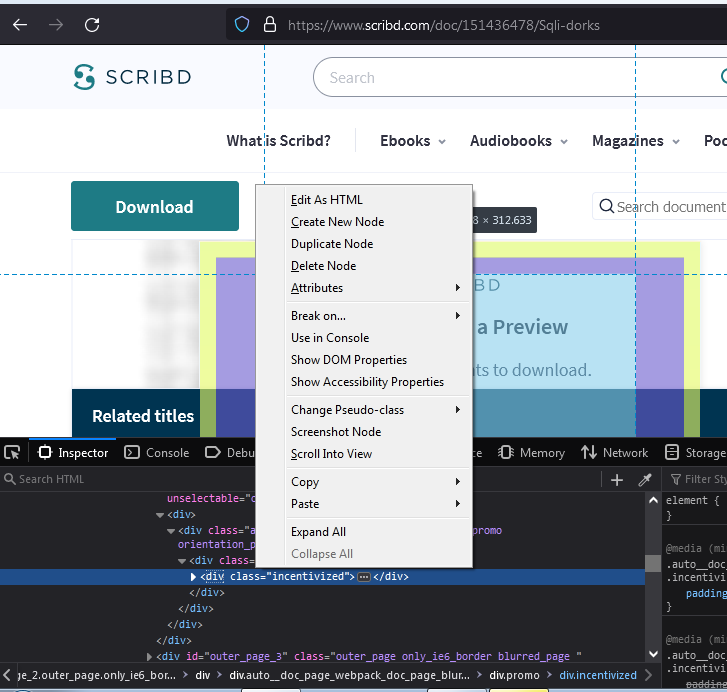The displayed image is a screenshot from the website Scribd.com. At the top of the webpage, there's a prominent search bar for user queries. Adjacent to the search bar are several tabs labeled "What is Scribd," "E-books" with a drop-down menu, "Audiobooks" with another drop-down menu, and "Magazines" also featuring a drop-down menu. Additional buttons on the interface include "Download," "Search Document," and "Related Titles."

In the middle of the image, a gray pop-up box is visible. This box contains a range of developer tool options such as "Edit as HTML," "Create New Node," "Duplicate Node," "Delete Node," along with attributes expandable via a right-facing arrow. Other options within the pop-up include "Break on" with a sub-menu, "Use in Console," "Show DOM Properties," "Show Accessibility Properties," "Change Pseudo Class" (expandable by another right-facing arrow), and actions like "Screenshot Node," "Scroll Into View," "Copy," "Paste" (each with further sub-menus), and the ability to "Expand All" or "Collapse All."

The background of the webpage is partially overlaid by the developer tool section, which emerges from the bottom. This section is black and features various tabs, including "Inspector," a partially obscured "Console" tab likely intended for debugging, "Memory," and navigation arrows for "Network," and "Storage." Below these tabs is a search function specifically for HTML code, followed by color-coded code snippets in black, blue, pink, purple, and white text.